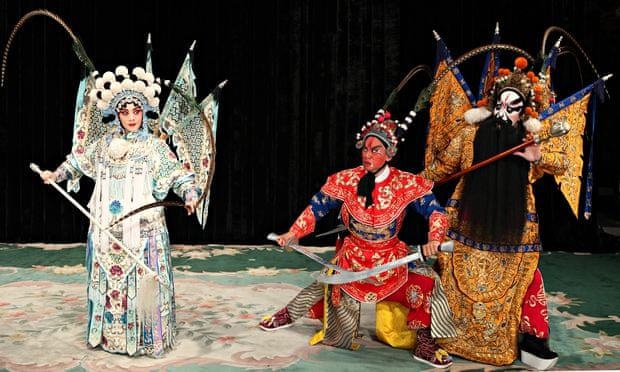This color photograph captures a dramatic kabuki performance on a richly decorated stage. On the left stands a woman in an elaborate white gown with intricate red, blue, and turquoise detailing. Her ensemble includes a large headdress adorned with black and white pom-poms and a striking structure of multicolored flags projecting from her back. She holds a sword in her right hand and gazes slightly to her right. In the center is an Asian man in a red tunic accented with red, blue, and white, his face painted with red markings. He is crouched down, holding two shiny silver swords in a defensive pose. On the far right, another man stands in a heavy-looking orange outfit, also displaying flags on his back. His face is painted with bold white and black designs, and he holds a walking stick topped with a gold knob. All three performers are positioned on a thick, ornate rug in shades of green, white, pink, and blue, against a black backdrop that intensifies the vivid colors of their elaborate costumes.